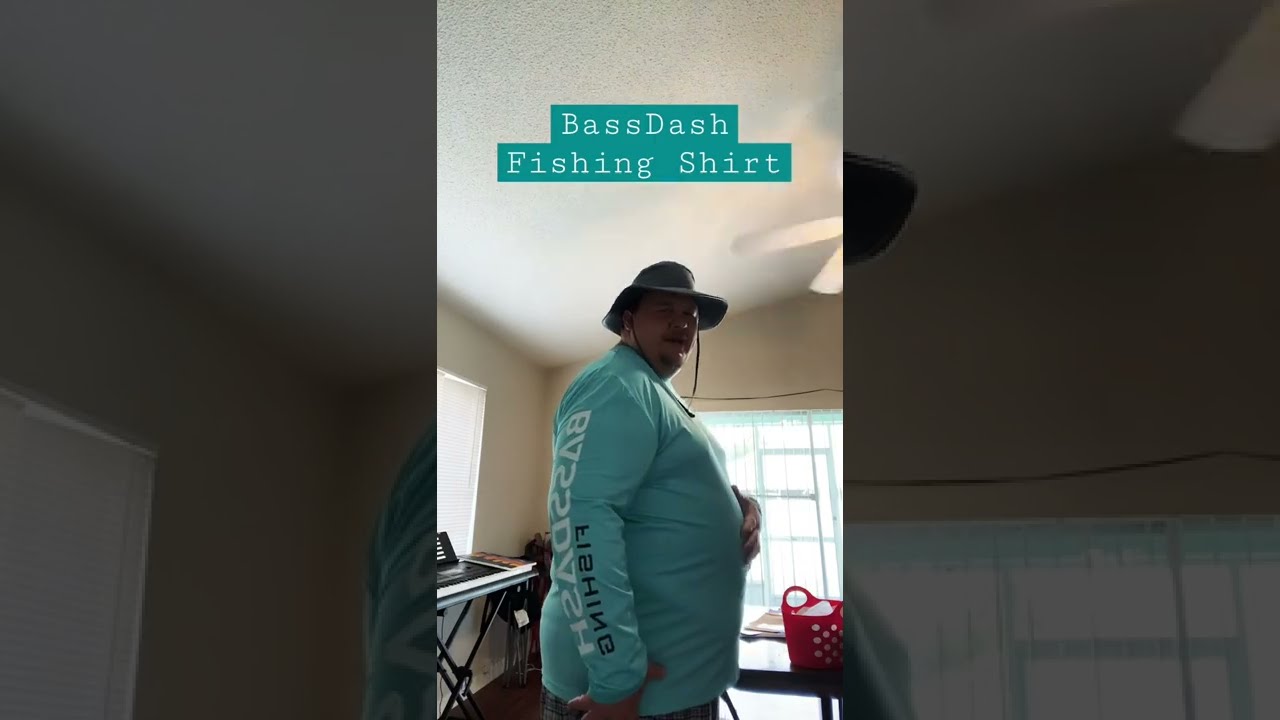The image, a screen capture from a social media video, is split into three sections, with the center displaying a large, heavyset man visible from the waist up. The man is facing to the right but looking straight ahead. He wears a gray hat with a black chin strap and a long-sleeve blue shirt that reads "Bass Dash Fishing" on the sleeve. The split image creates left and right segments that are zoomed-in portions of the center image with a dark filter. In the background are bright windows letting in natural light, a ceiling fan, a keyboard by one window, and a red basket on a table beside the man. The text "Bass Dash Fishing Shirt" appears in white font on a turquoise box above his head. The room has a white ceiling and various objects like a side table, adding to the setting.